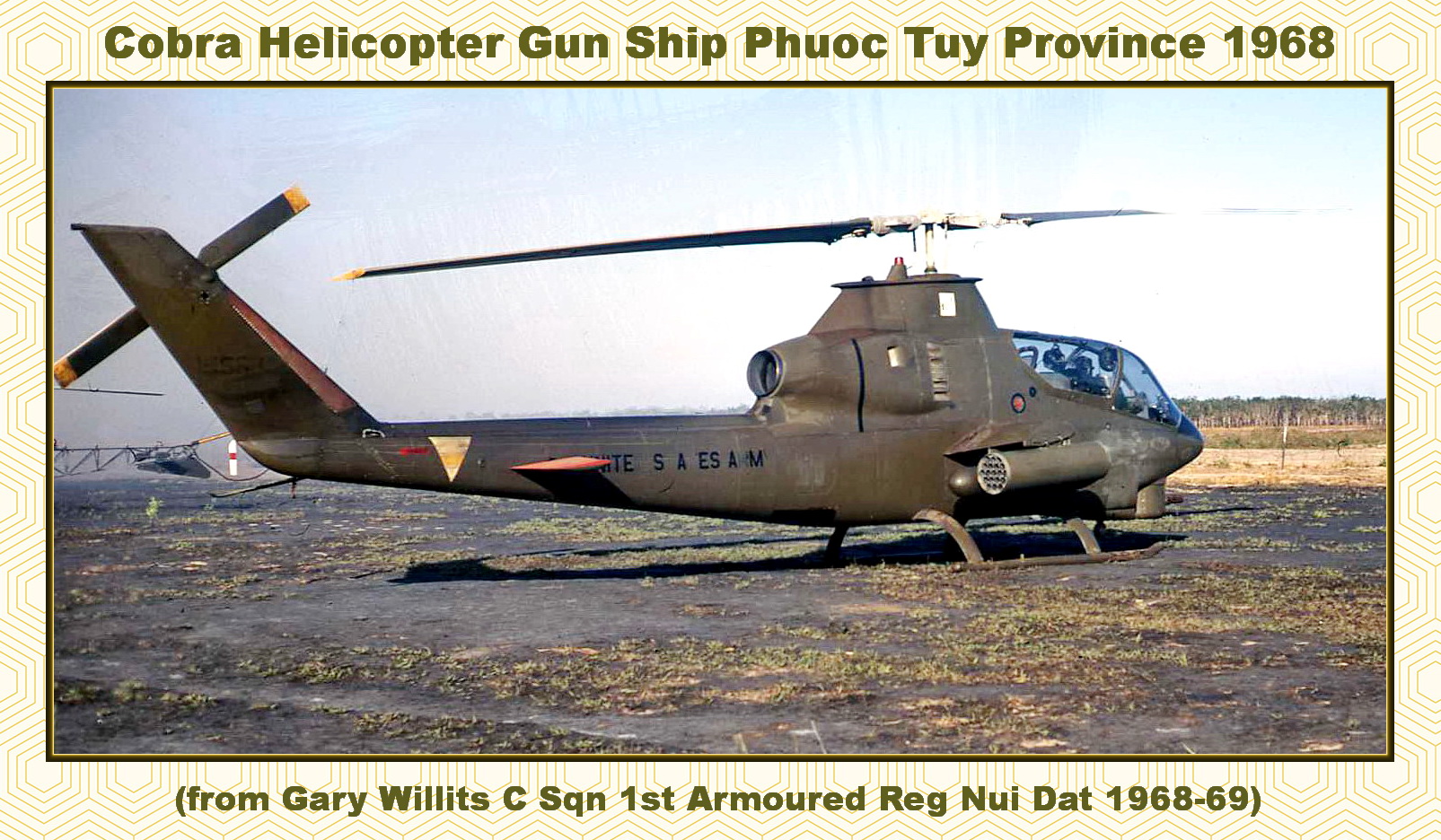The image prominently features a Cobra helicopter gunship centered in the photo, with its nose oriented to the right. Displayed above the helicopter is dark green text that reads, "Cobra Helicopter Gunship, Phuoc Thuy Province, 1968." Additionally, it includes, "from Gary Willits, CSQN, First Armored Reg, Nui Dat, 1968-1969." The helicopter is situated in the middle of a field, which contains what appears to be burned debris. In the background, another helicopter is visible, suggesting that this might be a common landing area for multiple aircraft. There is no clear indication of whether the helicopter belongs to Vietnam or the United States.